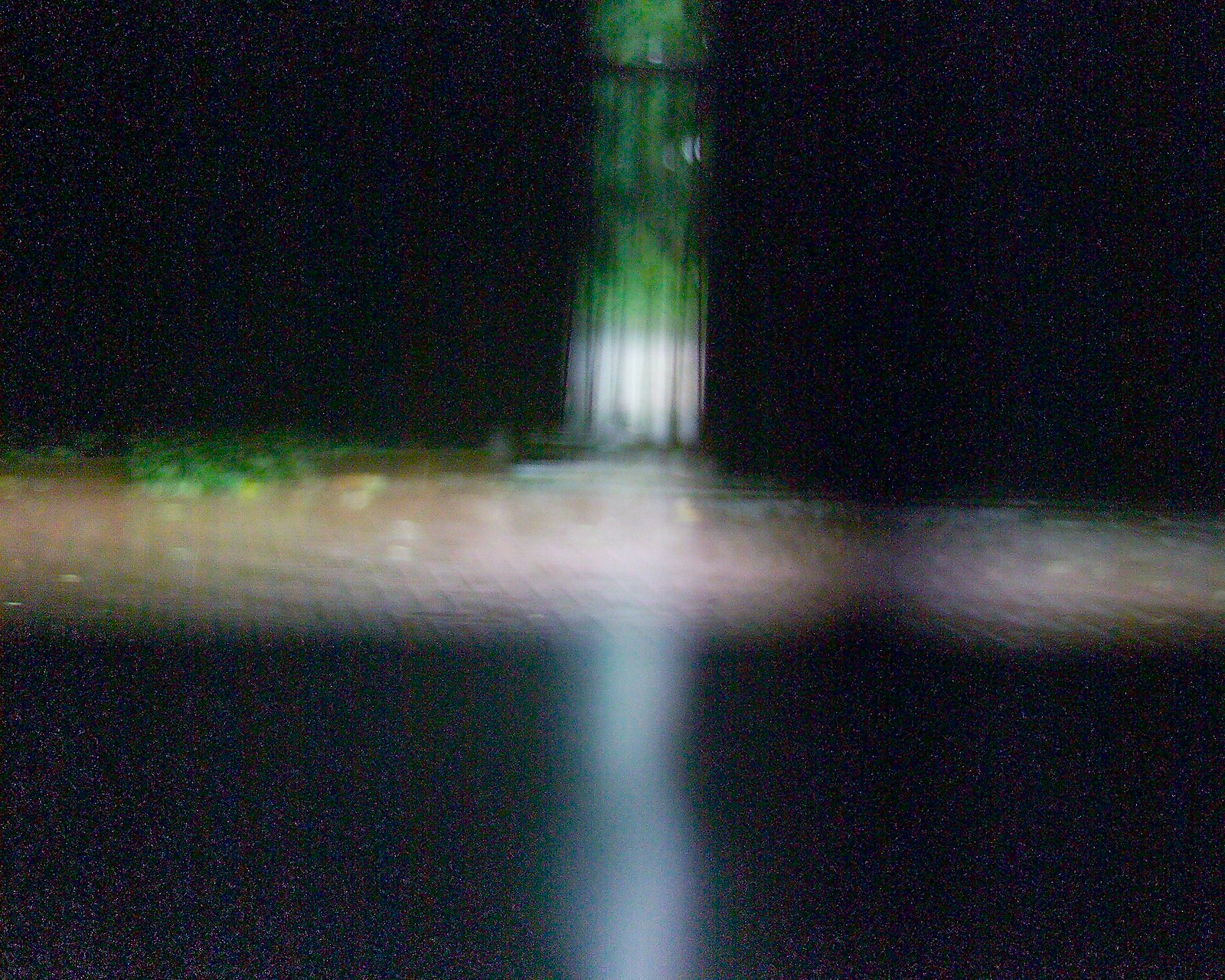The image depicts a dimly lit, barn-like structure shrouded in near-complete darkness. A singular beam of light penetrates through a narrow opening, illuminating a portion of the scene and providing a glimpse of the world outside. The external light reveals a verdant landscape with tall trees, suggesting an open, natural environment. Within the shadowy confines of the room, a reflective puddle of water hints at recent rainfall or a lingering downpour. Patches of green grass can be discerned amid the gloom, adding depth to the scene. A narrow fence is faintly visible, perhaps designed to allow small animals to pass through. The overall composition of the image captures the tranquil aftermath of rain, interspersed with subtle details indicating life and nature amidst the darkness.